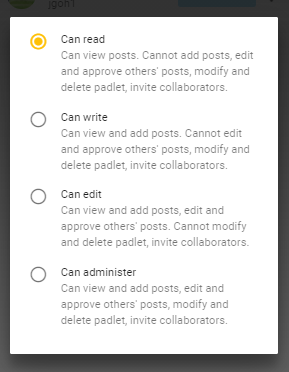The image features a prominently displayed white box set against a black background, which forms a frame around it. The white box contains four selectable options, each accompanied by a circle on the left side for selection. The first option is labeled "Can Read" and comes with a description stating "Can View Posts, Cannot Add Posts, Edit and Approve Others’ Posts, Modify and Delete Padlet, Invite Collaborators." This first option is checked and selected, causing the box around it to turn yellow, including the circle next to it. The second option is labeled "Can Write" and states "Can View and Add Posts, Cannot Edit and Approve Others’ Posts, Modify and Delete Padlet, Invite Collaborators." The third option is labeled "Can Edit," and the fourth and final option is labeled "Can Administer."